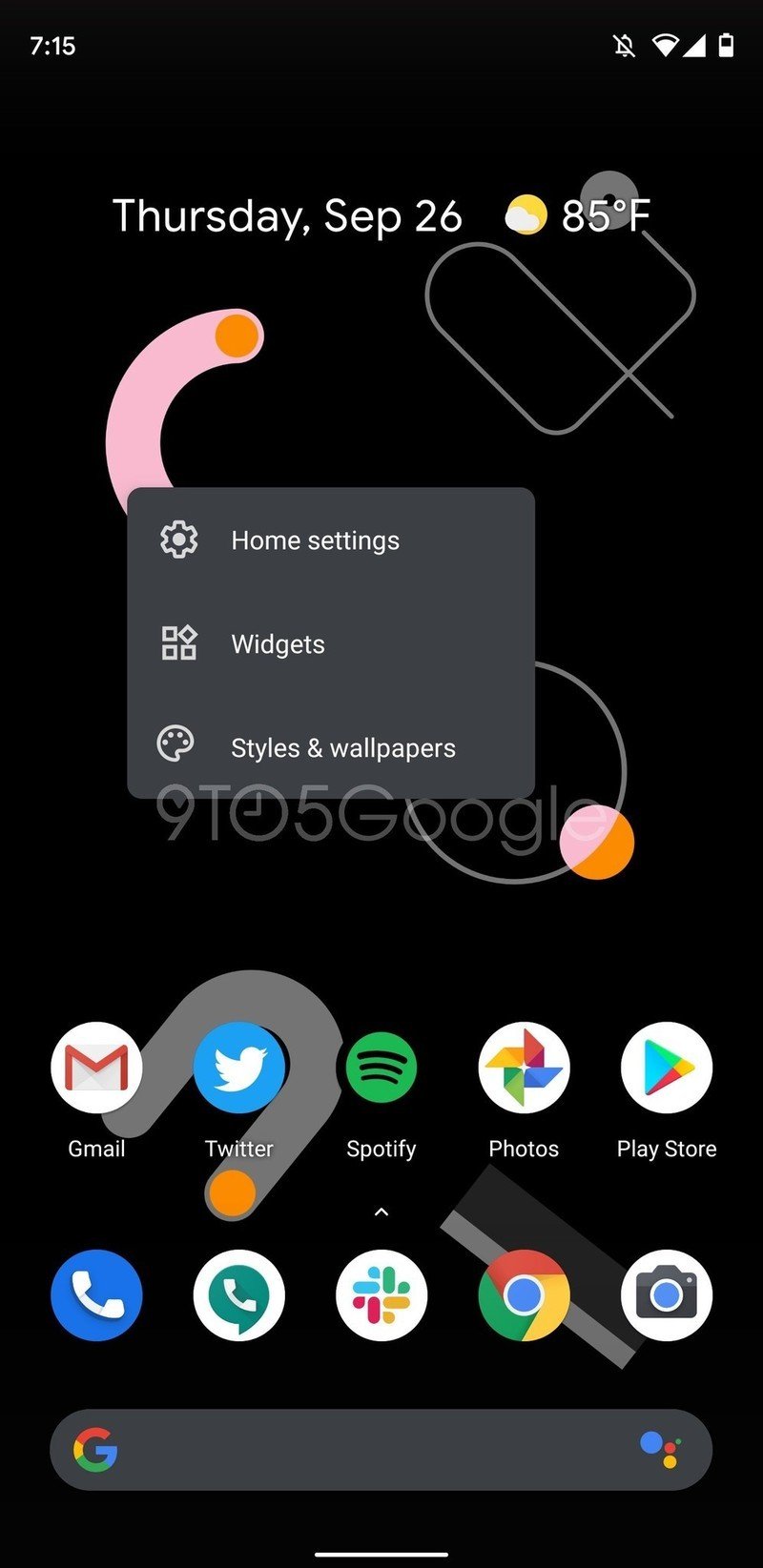The image is a vertically rectangular screenshot of a cell phone display. In the upper left corner, the screen shows the current time in white text as "7:15." Opposite this, in the upper right corner, icons indicate that the alarm is off and display the Wi-Fi, signal bars, and battery status. Centrally at the top, the date reads "Thursday, September 26," accompanied by the temperature, "85° Fahrenheit."

At the center of the screen, there is a pop-up window presenting a vertical list of options with corresponding icons for "Home settings," "Widgets," "Styles," and "Wallpapers." Faintly in the background, almost like a watermark, the text "9 to 5 Google" is visible.

At the bottom of the frame, two rows of app icons are displayed. The top row includes icons for Gmail, Twitter, Spotify, Photos, and the Play Store. The bottom row features icons likely for phone, text messaging (perhaps an additional photos app), Chrome, and the camera. Beneath these icons, in light gray text, is the Google search bar.